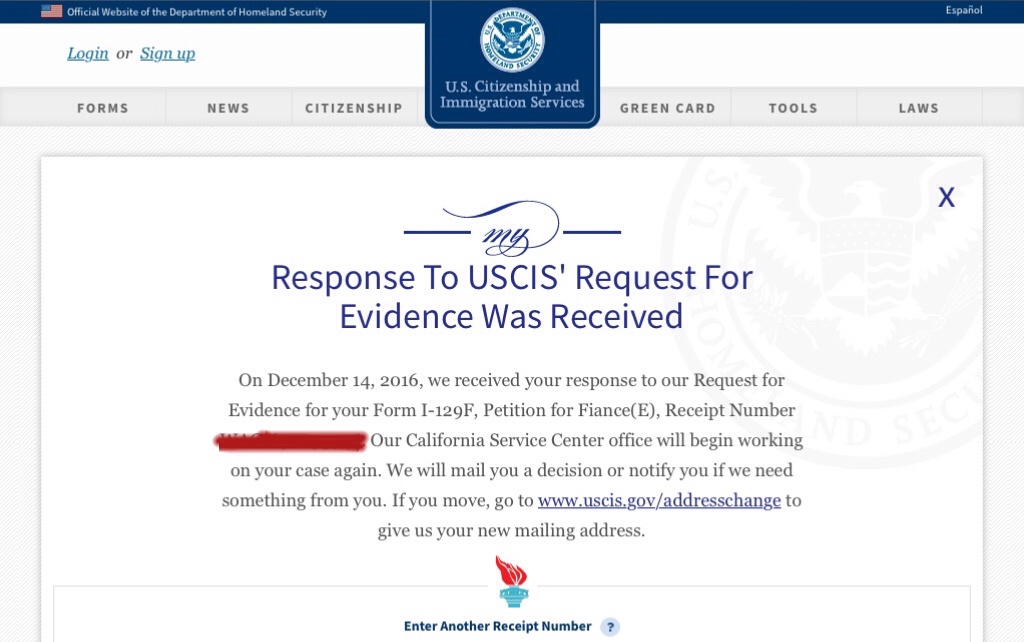The image features a prominent blue header with an American flag positioned on the left side. Adjacent to the flag, there is small, blue text that is difficult to read. Similar tiny blue text appears on the right side of the header. Below the header, a blue tab extends downward, partially overlaid by a gray rectangle that lists navigation options: "Forms, News, Citizenship, Green Cards, Tools, Laws."

At the center of the blue tab, a white circle contains an eagle emblem, surrounded by the text "U.S. Citizenship and Immigration Services." Beneath this section, a white rectangle with a gray outline is present, showcasing a formal notice. The notice reads in elegant script: "My response to USCIS," followed by "Request for Evidence was received."

The notification continues: "On December 14, 2016, we received your response to our request for evidence for your Form I-129F, Petition for Fiance." The E-receipt number has been obscured with red marker ink. It proceeds to state: "Our California Service Center office will begin working on your case again. We will mail you a decision or notify you if we need something from you. If you move, go to [website URL in blue] to give us your new mailing address."

Finally, the image features a depiction of a blue torch with a red flame. Below the torch, it reads "Enter another receipt number" in blue text. Adjacent to this, there is a blue circle containing a darker blue question mark.